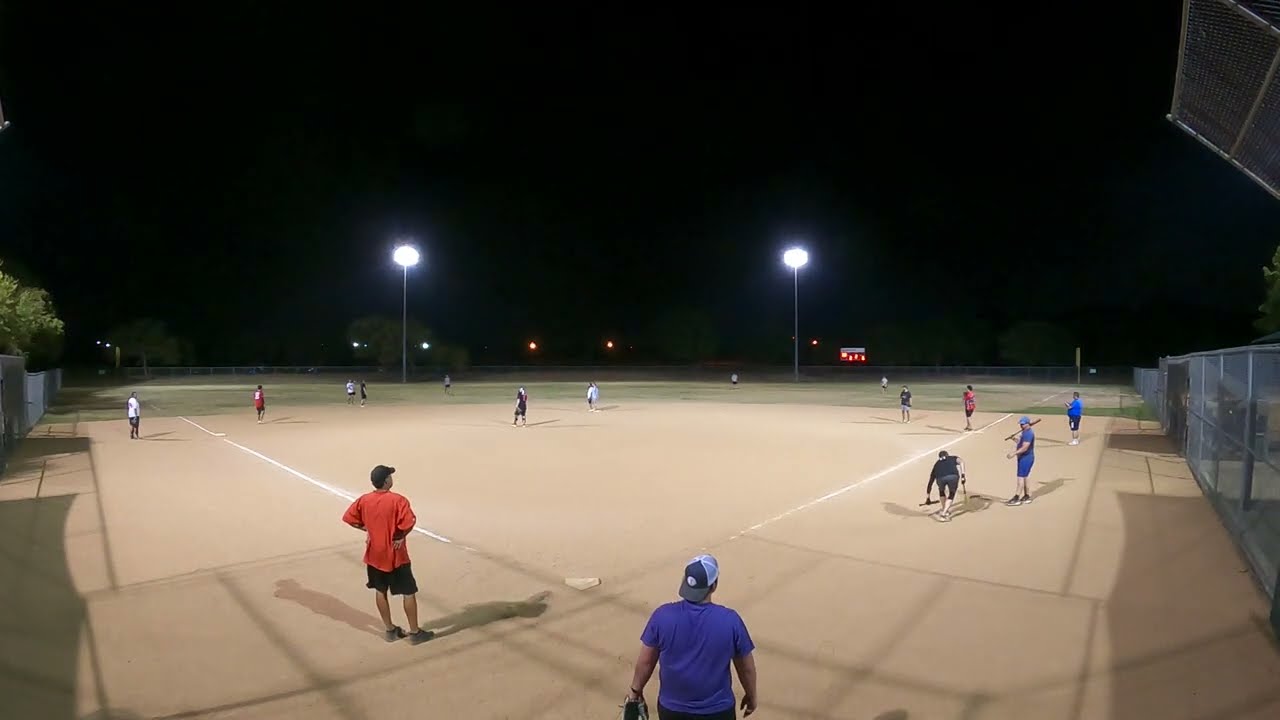This nighttime photograph captures a recreational baseball game played by middle-aged men wearing various colored t-shirts—primarily red, blue, white, and black—and shorts, rather than uniforms. The shot is taken from behind home plate, offering a full view of the inky black sky illuminated by two large stadium lights positioned behind the outfield on the left and right, creating a well-lit field. The tan, sandy playing field is outlined by white painted lines and is surrounded by a fence that runs from the right side around the entire field. In the background, there are a few small trees and a distant scoreboard with red lights and a white top, though the numbers are not visible. The players are spread out in their respective positions, with no one currently at bat. To the left of home plate, a man in an orange shirt stands, possibly serving as an umpire or waiting for his turn to play. The scene includes the batter, pitcher, and catcher, with most of the players standing in the sandy infield while the grassy outfield stretches behind them.